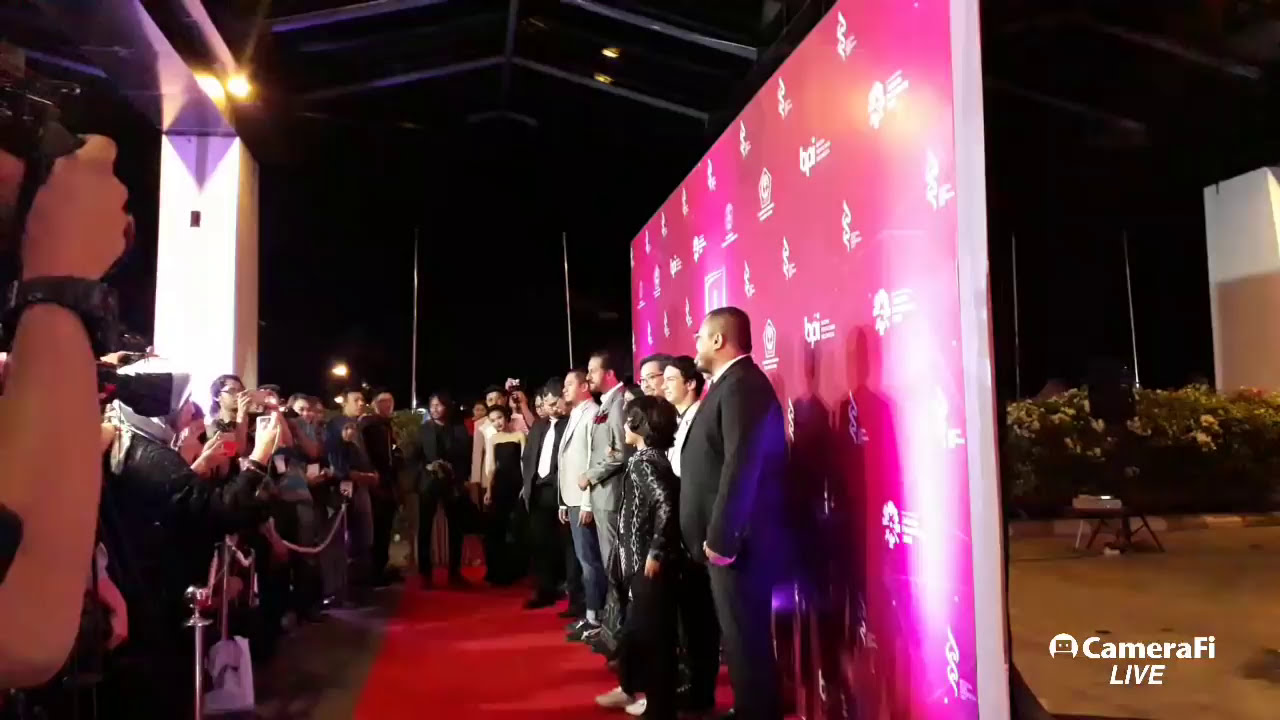This horizontally aligned rectangular image captures an outdoor red carpet event at night, evidently a press photo op covered via CameraFi Live as indicated by the logo in the bottom right corner of the photograph. Central to the scene is a partition wall draped in a pinkish-purple backdrop adorned with various white logos, designed to ensure branding is visible in photo frames. Positioned before this decorative partition, a group of seven to eight individuals, including what appears to be actors or musicians dressed in formal attire, stand posed for photos. The ensemble includes men in suits, a woman in a long black dress, and a young boy in a shimmering jacket. The event space itself is roped off, with members of the press huddled on the other side, busily snapping pictures with cameras and phones. To the right of the partition wall, flowers are visible, contributing to the aesthetic environment supported by steel framework overhead that forms a ceiling. Behind the wall, a hedgerow adds to the outdoor ambiance of the event.